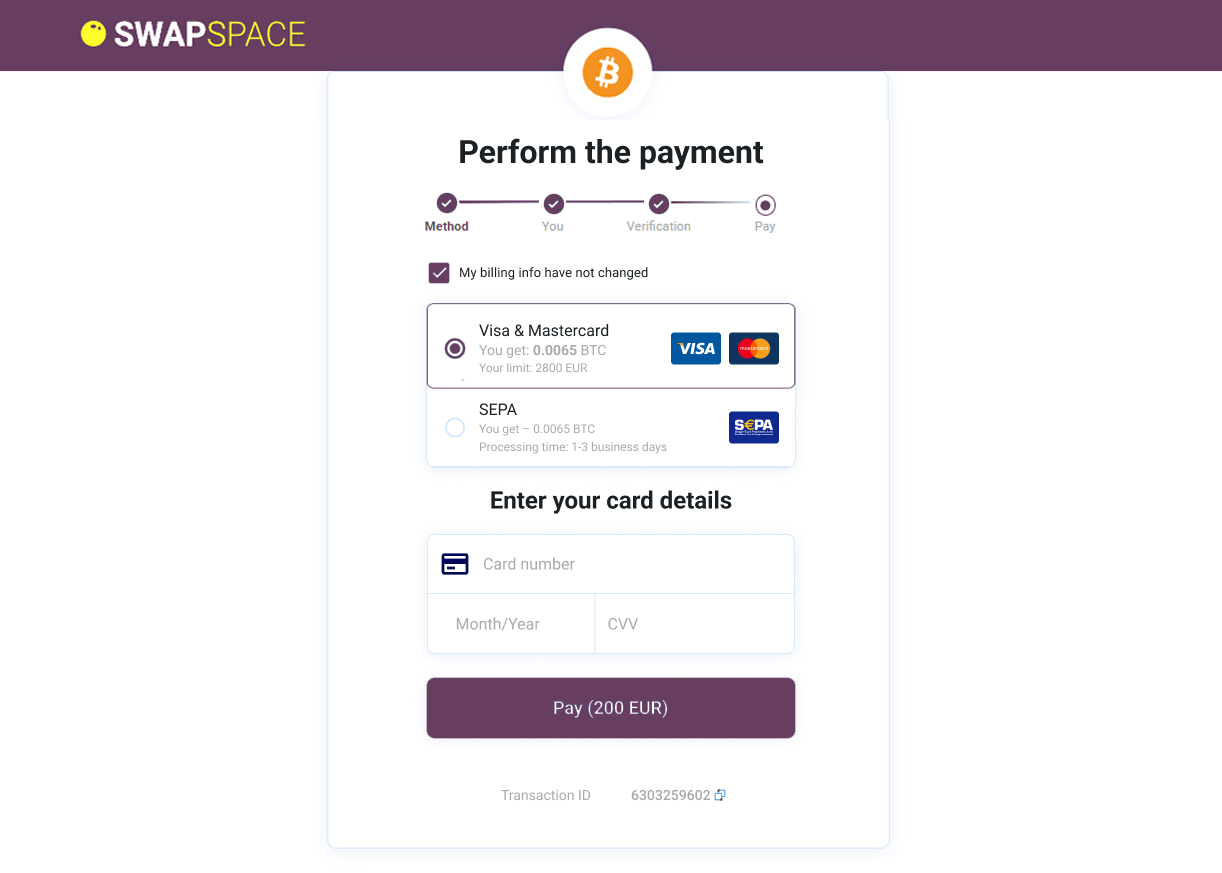This is a screenshot from the SwapSpace platform, illustrating the payment process. In the upper left corner, the "SwapSpace" logo is prominently displayed. The word "Swap" is in bold white font, while "Space" is in thin, all-capitalized yellow letters. A yellow circle sits to the left of the logo, all nestled within a purplish horizontal bar that spans the width of the screen.

At the center of this purple bar, there's a white circle with an orange circle inside it, featuring the Bitcoin logo. Below this bar, the main payment section is visible. It includes a status bar indicating the stages of the payment process: "Method," "Verification," and "Pay." Both the "Method" and "Verification" steps are marked as completed with checkmarks.

Underneath the status bar, there is a checkbox labeled "My billing information has not changed," which is checked. The payment method selected is Visa/MasterCard. Finally, at the bottom center of the screen, there is a large "Pay €200" button, indicating the amount to be paid.